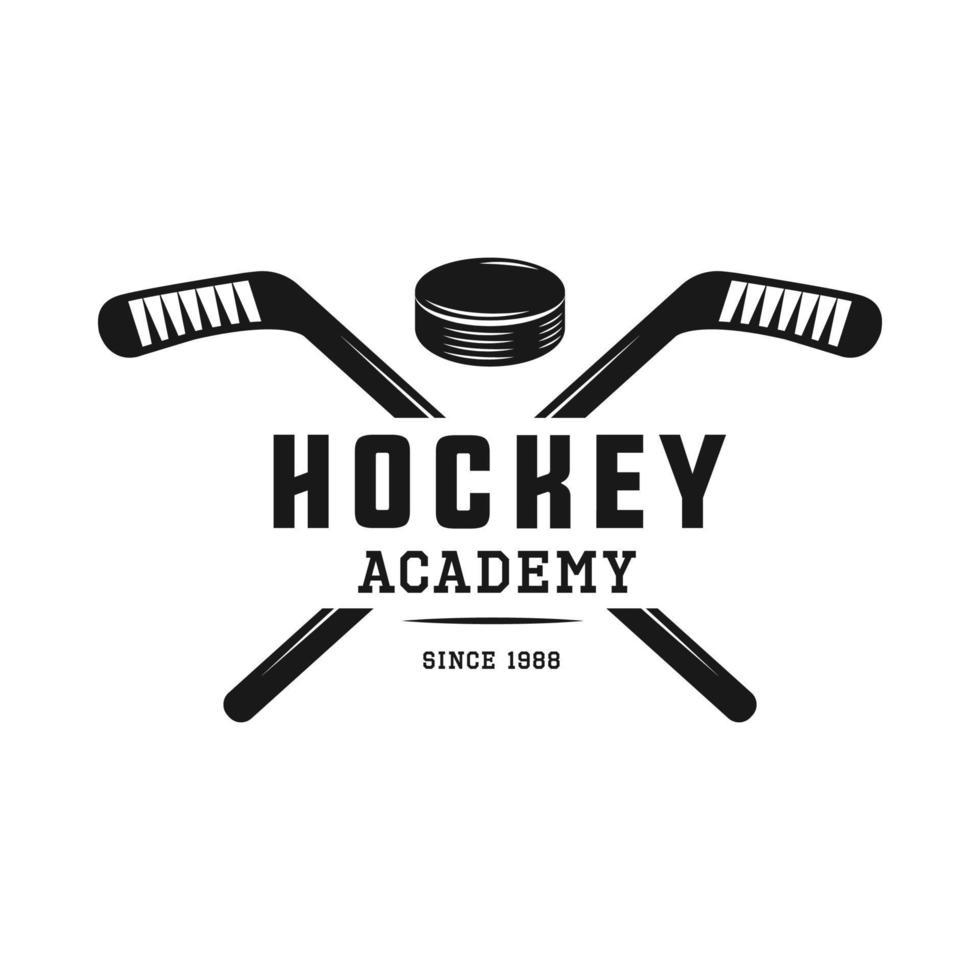The image is a black and white logo for a Hockey Academy established in 1988. The background is pure white, and at the center, a pair of black hockey sticks form an X-shape, with their handles at the bottom corners and their blades at the top corners. The blades feature white stripes that look like hockey tape wrapped around them. Between the crossed sticks, near the top, is a black hockey puck detailed with white lines to give it dimension. At the center of the logo, bold black text reads "HOCKEY ACADEMY" with "Since 1988" written directly beneath it. The text is in uppercase and clearly stands out against the white background.